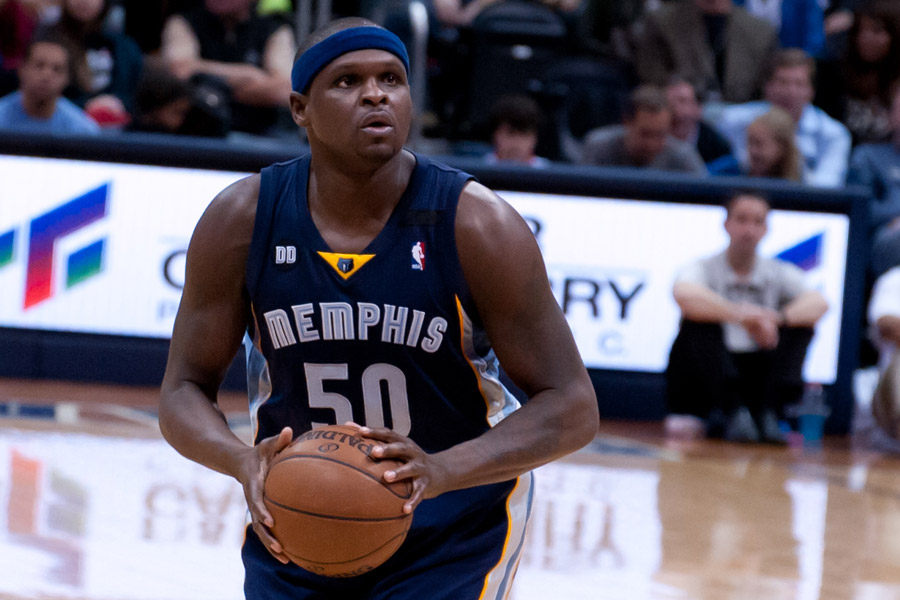The photograph captures an intense moment with a basketball player, presumably from the Memphis Grizzlies, positioned on an indoor basketball court. The court's highly reflective, polished, light brown wooden flooring is marked with various white lines indicating areas of play. The player, a black man with closely shaved hair, is dressed in a sleeveless blue NBA jersey featuring the word "Memphis" and the number 50 in white, complemented by yellow and white stripes along the sides. He has a blue sweatband around his head and is holding a brown leather basketball with both hands, looking upward, likely towards the basket, with a focused expression. Behind him, a tiered seating area is packed with spectators sitting on black fold-up seats. A white banner with partially obscured black letters hangs from the short wall separating the audience from the court. The blurred background also includes a few individuals seated near the banner, adding to the dynamic atmosphere of the scene.